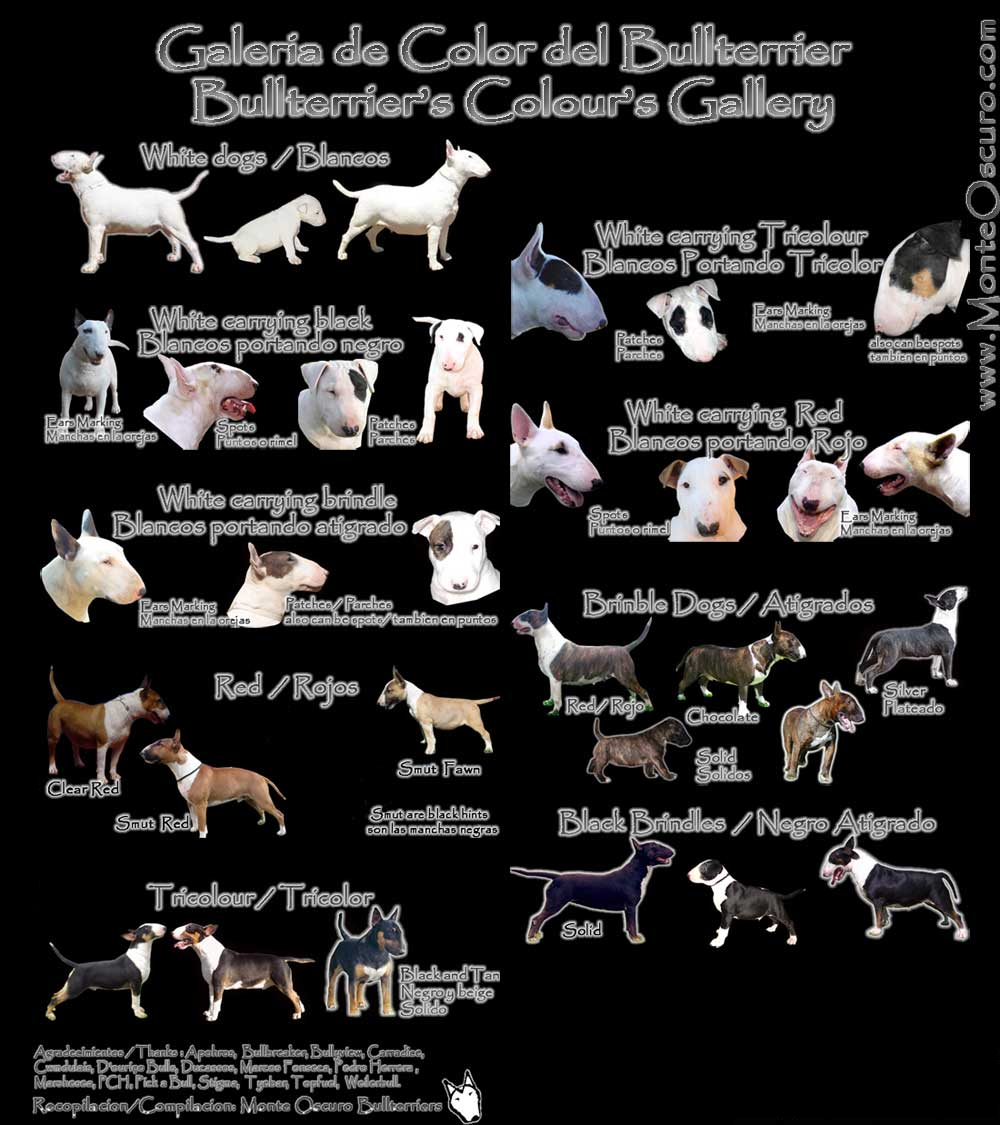The photograph showcases the "Galleria de Color del Bull Terrier" or "Bull Terriers Colors Gallery," set against a black background. The exhibit is bilingual, presenting descriptions in both English and Spanish. Displayed are multiple images of Bull Terriers organized by color categories. 

- **White Dogs (Blancos)**
  - Pure white Bull Terriers.
- **White Carrying Black (Blancos Portando Negro)**
  - White Bull Terriers with genetic markers indicating black coloration.
- **White Carrying Brunel (Blancos Portando ...)**
  - Although slightly blurred, this refers to white Bull Terriers carrying Brunel (likely a typo for brindle) genes.
- **Red (Roja)**
  - Bull Terriers with a red coat.
- **Tricolor (Tricolor)**
  - Bull Terriers with tricolor patterns.
- **White Carrying Tricolor (Blancos Portando Tricolor)**
  - White Bull Terriers with tricolor genes.
- **White Carrying Red (Blancos Portando Rojo)**
  - White Bull Terriers carrying red coloring genes.
- **Brindle Dogs**
  - Bull Terriers with a brindle coat.
  - **Black Brindle (Negro Brindle)** - Described as 'affogatos' in a mixture of both black and brindle patterns.

Each category is visually represented with photographs displaying the respective Bull Terrier color variations. Additional details include the website "www.montiasquiro.com" located on the upper right side and a small, unreadable text with a dog head logo in the bottom left corner of the image.